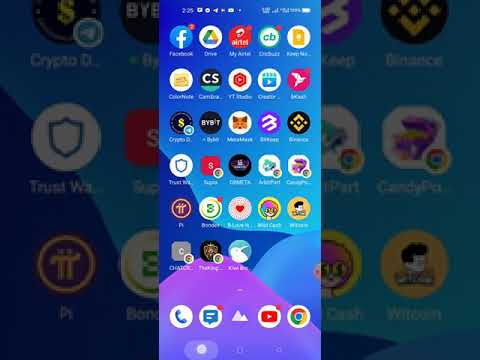The image depicts a low-resolution, compressed screenshot of an Android phone's app tray, centrally placed within the frame, featuring numerous rounded app icons. The focal point is a close-up of the app icons, which are overlaid on a dark, blurred background displaying an enlarged, grayed-out version of the same icons. The home screen, dominated by a variety of apps, is set against an abstract wallpaper with overlapping blobs—purple at the bottom, blue to the right, and a large light-blue transitioning to deep blue at the top.

Notable app icons include familiar utilities and browsers such as Facebook (blue and white), Google Drive (yellow, green, and blue), YouTube (red and white), and Google Chrome. There are also several game apps, including "Candy Pig" and "Pie," alongside other applications like Bytebit and a potential security app depicted by a shield icon. Additional icons visible are a white bird on a red background, a movie logo with a play button, a money sign on black, and various colorful symbols. The bottom of the screen showcases a distinct navigation bar with common Android controls: a circle, a square, and another unspecified button.